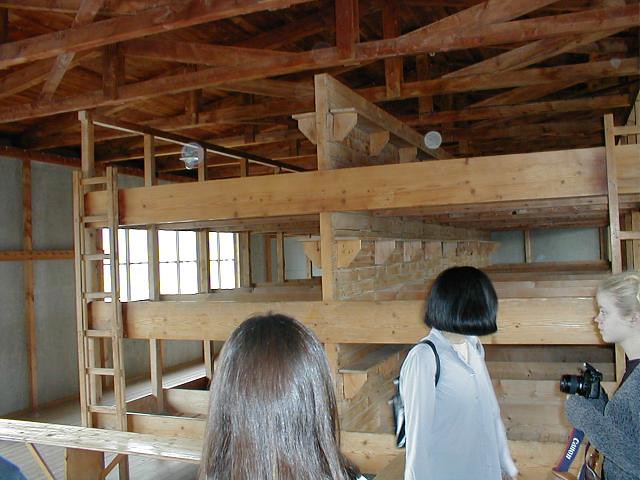The photo depicts an industrial-looking building with wooden beams overhead and numerous light fixtures hanging down. In the background, there are several rows of bunk beds, each fitted with a ladder, arranged in a grid-like pattern. The bunk beds are bare, devoid of comforters or any bedding. The brick and wooden walls add a rustic charm to the room.

In the foreground, three young women are present. The central figure, whose back is facing the camera, has straight brown hair. To her right, a girl with a bob cut of straight black hair is seen wearing a white button-up shirt paired with a small black backpack. On the far right, another girl, with her hair tied up, is holding a camera and is dressed in a gray long-sleeved sweater. The space between the wooden separators almost gives the impression of animal stalls, but it's clear they are instead empty bunk beds. The women seem to be observing and possibly exploring this unique, minimalist environment.